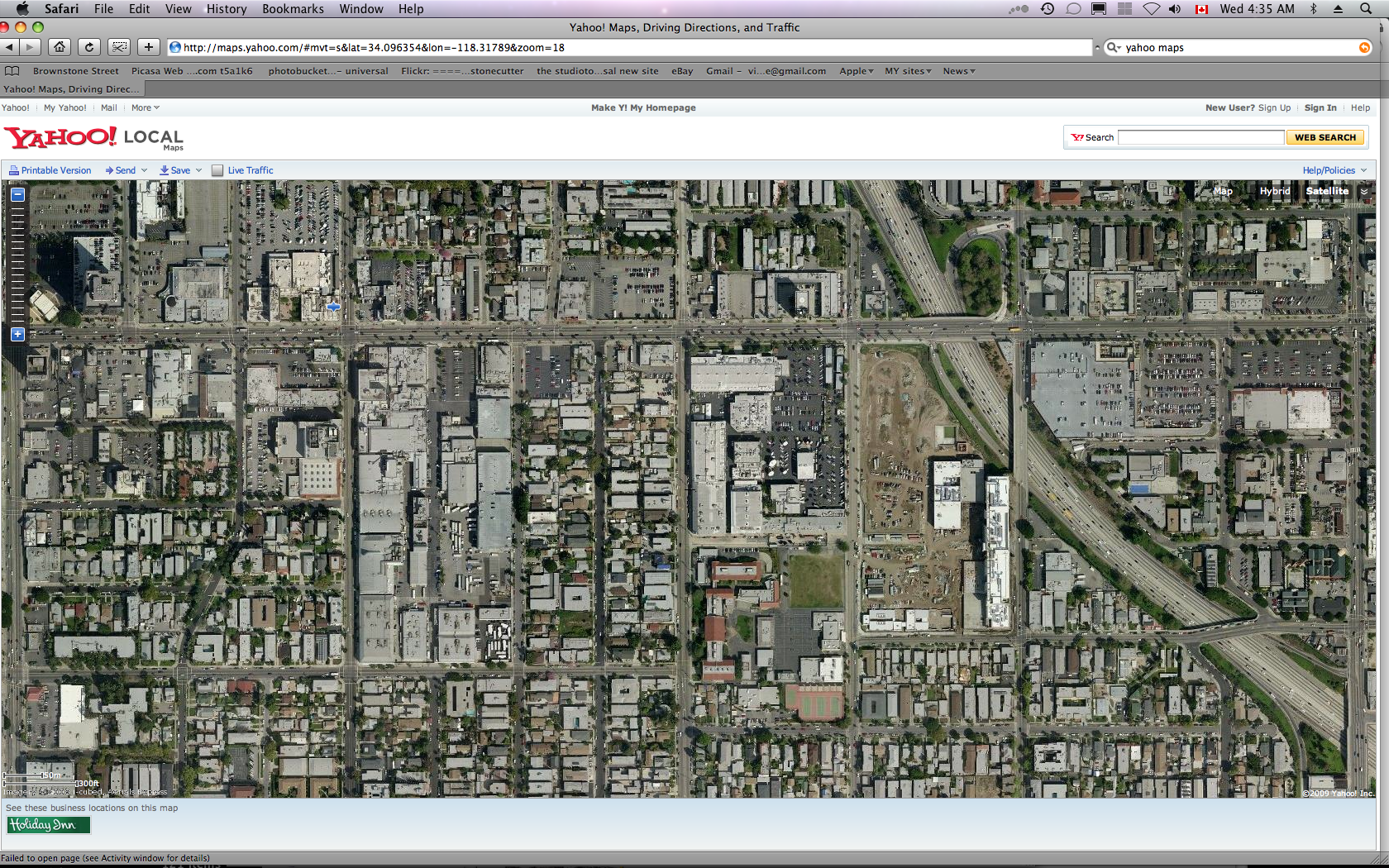The image appears to be a printout of an aerial view of a city on Yahoo Local Maps. Predominantly gray with numerous rectangular shapes indicative of buildings, the cityscape also features a highway running along the right side. Scattered throughout are pockets of green, possibly parks or other green spaces, and a brown area that seems to be an empty lot or dirt pit without direct highway access. The highway itself is a major thoroughfare, with at least four lanes in each direction, highlighting its significance and busyness.

In the upper center portion of the image, there's a city block with a notable mixture of building sizes and a large parking area. One long building and three smaller ones occupy a considerable portion of this block. Additionally, a sideways building spans about two-thirds the length of the three smaller buildings. Two more small buildings and a small long building also populate this area, with the remaining space dedicated to parking.

Due to the limitations of the image resolution, it is difficult to ascertain the specific functions or details of the roofing on these buildings. The smaller structures could be residential houses, apartment buildings, or other small establishments. The brown area adjacent to the highway resembles a dirt pit or undeveloped land, and the highway itself is a limited access road, emphasizing its role as a major transit route.

Overall, the image depicts a densely built city with a mix of commercial and residential areas, significant green spaces, and a substantial transportation network.